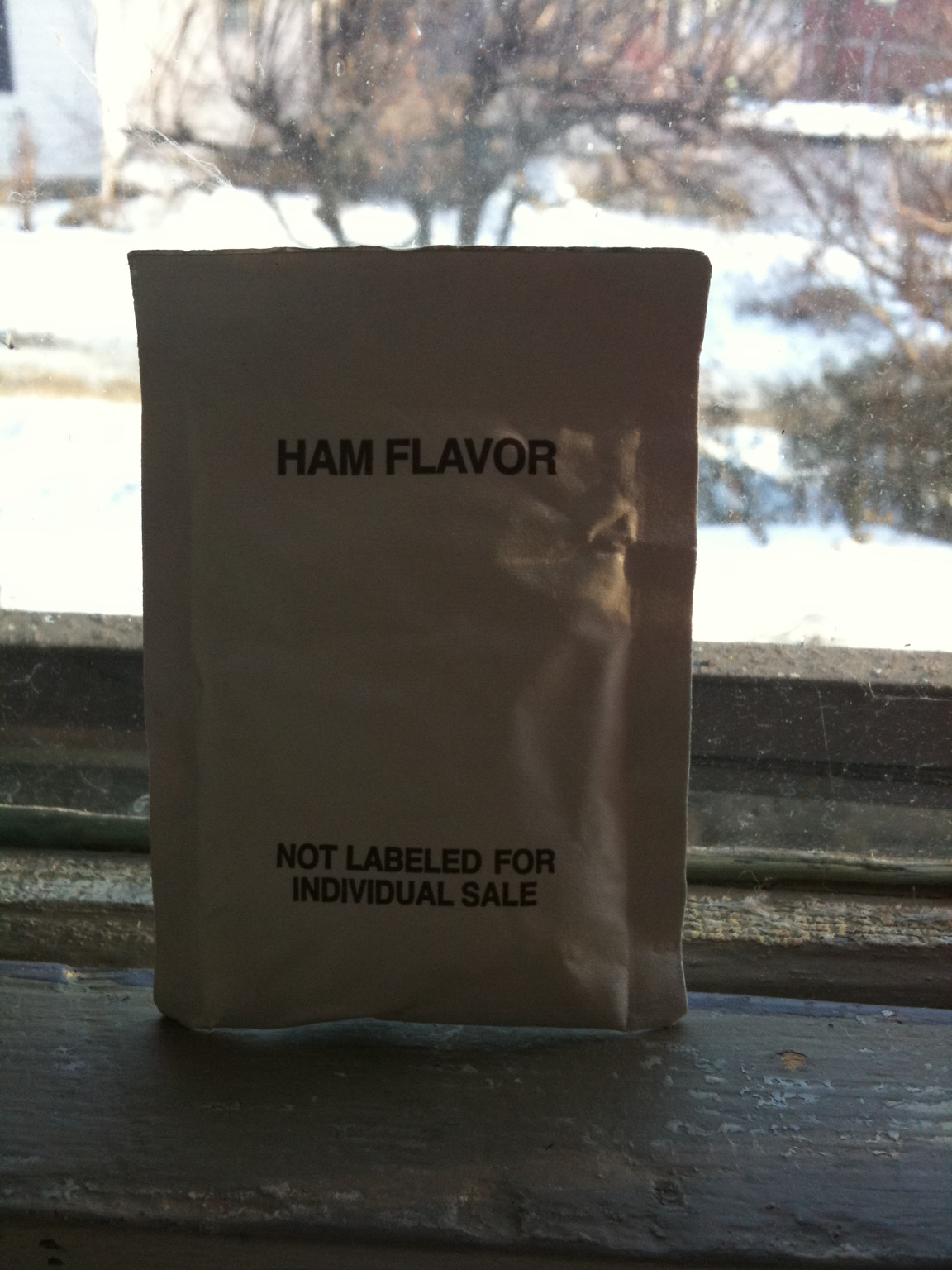The image depicts a color photograph of a white, rectangular plastic packet standing upright on a wooden windowsill. The packet, reminiscent of an Army MRE (Meal Ready-to-Eat), has the text "ham flavor" written in black font, along with the note "not labeled for individual sale." The windowsill appears to be painted a grayish blue. Beyond the single-pane wooden window, the out-of-focus background reveals a snowy landscape featuring a leafless tree, a substantial blanket of snow, and a distant building. The scene captures an indoor moment, contrasting the warm wooden tones with the cold, snow-covered outdoors.